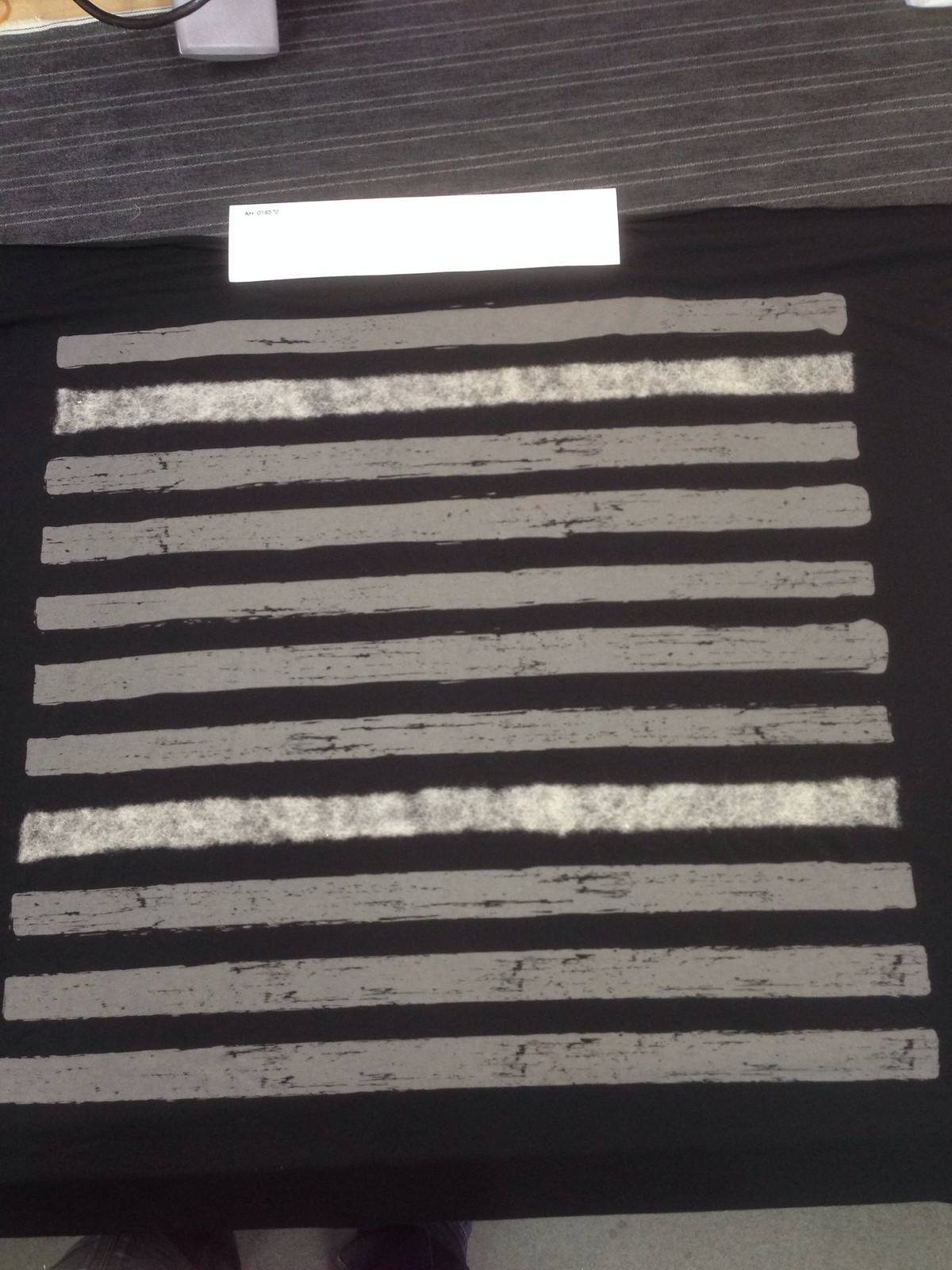This detailed description can be refined as follows:

---

A meticulous photograph captures an intriguing art piece executed on a black substrate, which could either be construction paper or a sheet from a sketchbook. The artwork is affixed to its background using a strip of white tape at the top edge. The backdrop against which the piece is mounted features a pattern of gray and light gray stripes.

The central composition of the piece itself comprises several horizontal lines, characterized by their thick, rectangular shapes. The colors of these lines range from light gray to a lustrous silver, with varying shades of gray interspersed in between. There is no discernible pattern or sequence in the arrangement of these colors, giving the piece a spontaneous and abstract quality. 

Additionally, the artwork exhibits a textured surface, suggesting a potential portrayal of a wooden fence with the lines representing slats. The deliberate yet random distribution of colors and textures invites viewers to engage deeply with the piece, sparking interpretations that may extend beyond the initial impression of a simple depiction.